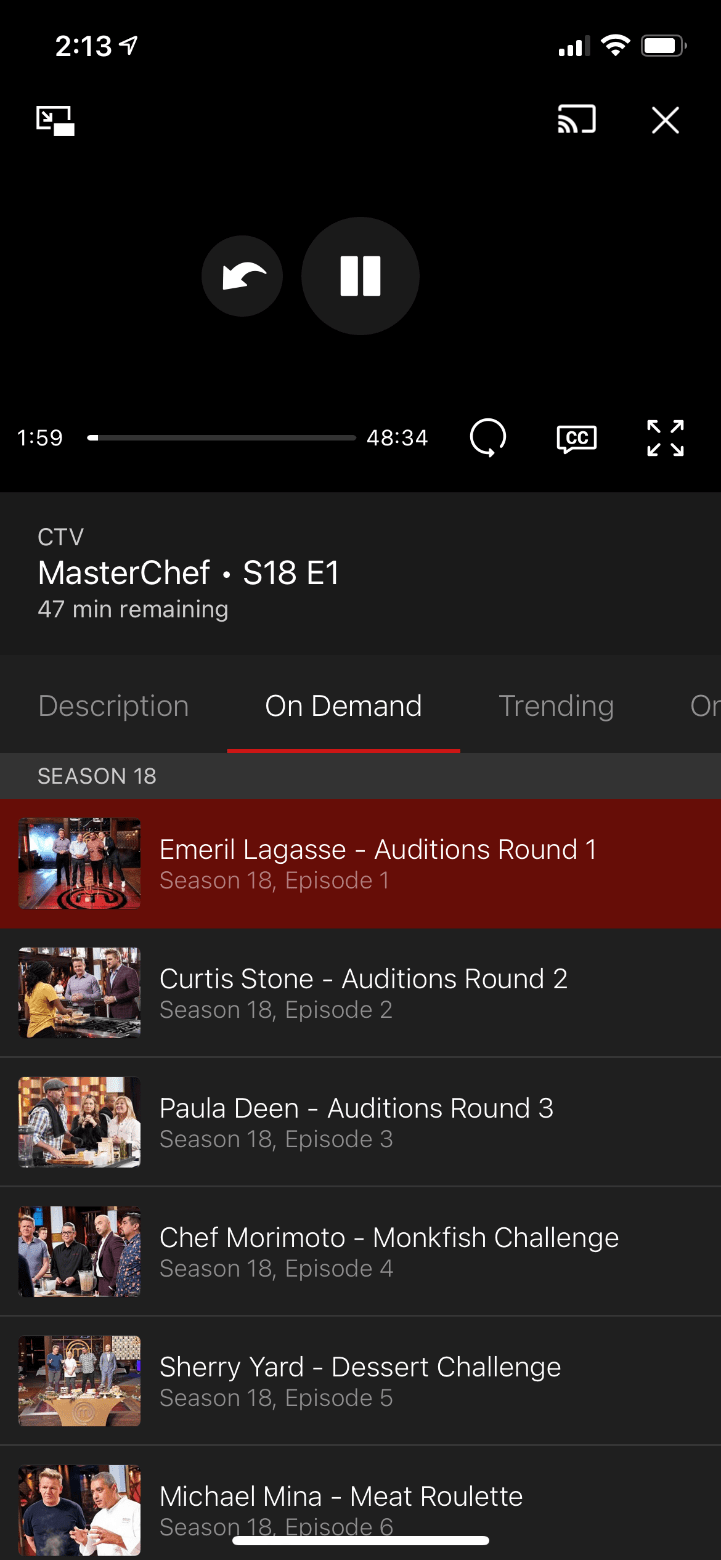The image shows a paused video on a mobile app, with the timestamp frozen at 1 minute and 59 seconds. The total duration of the video is 48 minutes and 34 seconds, and 47 minutes remain. The currently playing video is an episode of Masterchef, specifically Season 18, Episode 1. The screen displays three main tabs: Description, On Demand, and Trending, with a partially cut-off fourth tab. The "On Demand" tab is highlighted with a red line underneath it, showcasing other episodes from Season 18. The top of the screen indicates that the current episode features "Emeril Lagasse Audition Round One," marked in red to show it is the active episode. Below this, thumbnails and titles for other episodes in Season 18 are visible, listing episodes 1 through 6.